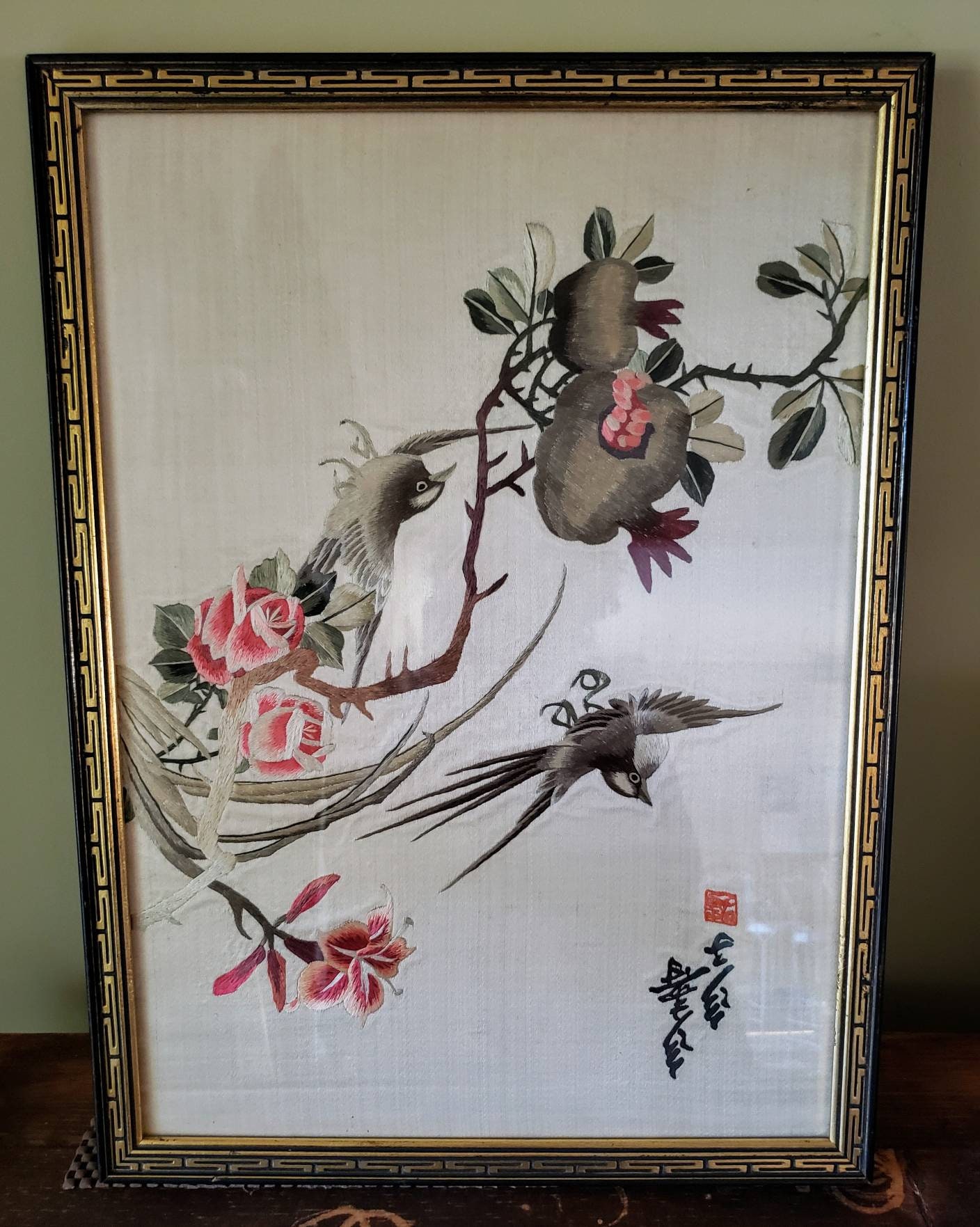The picture showcases an elegantly framed painting resting on a dark brown wooden table. The frame, crafted with a gold outline featuring a consistent square-like design, encloses a delicate fabric piece with an intricate, traditional design. The painting itself has a subtle gray background and prominently features a detailed botanical scene. A branch extends upward towards the left, adorned with two red roses with pink outlines, accompanied by another flower resembling a lily with white outlines and red accents. The brown branch supports two gray fruits capped with purple buds, surrounded by a mix of white, light green, and dark green leaves. A pink worm is seen emerging from one of the fruits.

Two birds are depicted in the scene: one, black, white, and gray, is flying up towards the fruit from below, while the other, predominantly black and dark gray with hints of white, appears to be flying upside-down near the fruit on the right side. At the base of the painting, two vertical autographs in black text sit next to a red emblem, with Chinese or Japanese characters written along the right side. The overall composition, rich in detail and various shades of black, gray, pink, and green, captures a serene and dynamic interaction of nature.